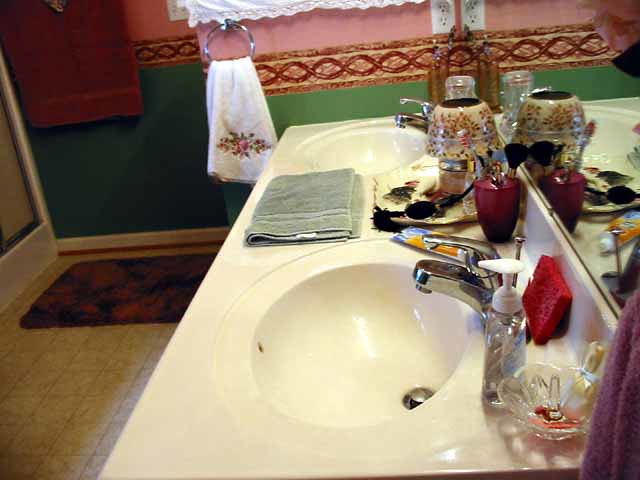Looking down the length of a modern vanity, this bathroom setup features two integrated oval-shaped sinks molded seamlessly into a smooth, white plastic countertop. A matching molded backstop runs the length of the countertop, providing a cohesive look. Each sink is equipped with a sleek, silver, single-handle faucet. Between the sinks, a neatly folded gray towel lies beside a small, undefined tray containing miscellaneous items that are slightly out of focus.

In the foreground, a glass dish with a central pillar, likely intended for holding rings while washing, stands next to a clear bottle of liquid soap with a pump top. Behind the fixture of the front sink, a red sponge is also visible. Adding a touch of color and storage, there is a covered container in a rich, dark red hue that gradients to black towards the bottom, its content unspecified. A large ceramic vase, devoid of flowers, boasts a gray glaze with a delicate floral pattern near the back.

Dominating the wall behind the sinks is an expansive mirror reflecting the room's details. The lower portion of the room's walls is painted a soothing green, transitioning to a pink hue above a decorative wallpaper border. Affixed to the wall is a silver towel ring holding a white towel adorned with an embroidered floral pattern, and nearby hangs a brown towel.

To the side, there is a glimpse of a shower enclosure with a glass door. The floor is covered in light brown tiles, providing a warm base, and a dark black bath mat with a subtle dark red floral pattern lies underfoot, completing the inviting and functional bathroom space.